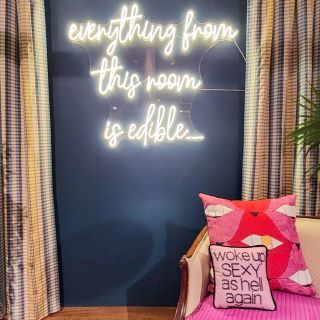This indoor photograph, approximately two inches square, captures a colorful and detailed scene. The background features a window adorned with vibrant striped curtains, composed of various colors including grey, pink, orange, black, and hues of light blue, yellow, pink, and purple, arranged in a crisscross pattern of thinner stripes. In the center of the image, a black area highlights a bright, white cursive text that reads, “everything in this room is edible,” illuminated as a sign. To the right, beneath the window and curtains, is a corner of a low-backed chair with a wooden armrest. Atop the chair, there are two pink pillows; the smaller pillow has playful teeth details, while the larger one is adorned with the black, bold text, “woke up sexy as hell again.” The pillows, especially the one with the text, effectively complement the whimsical message presented in the image.